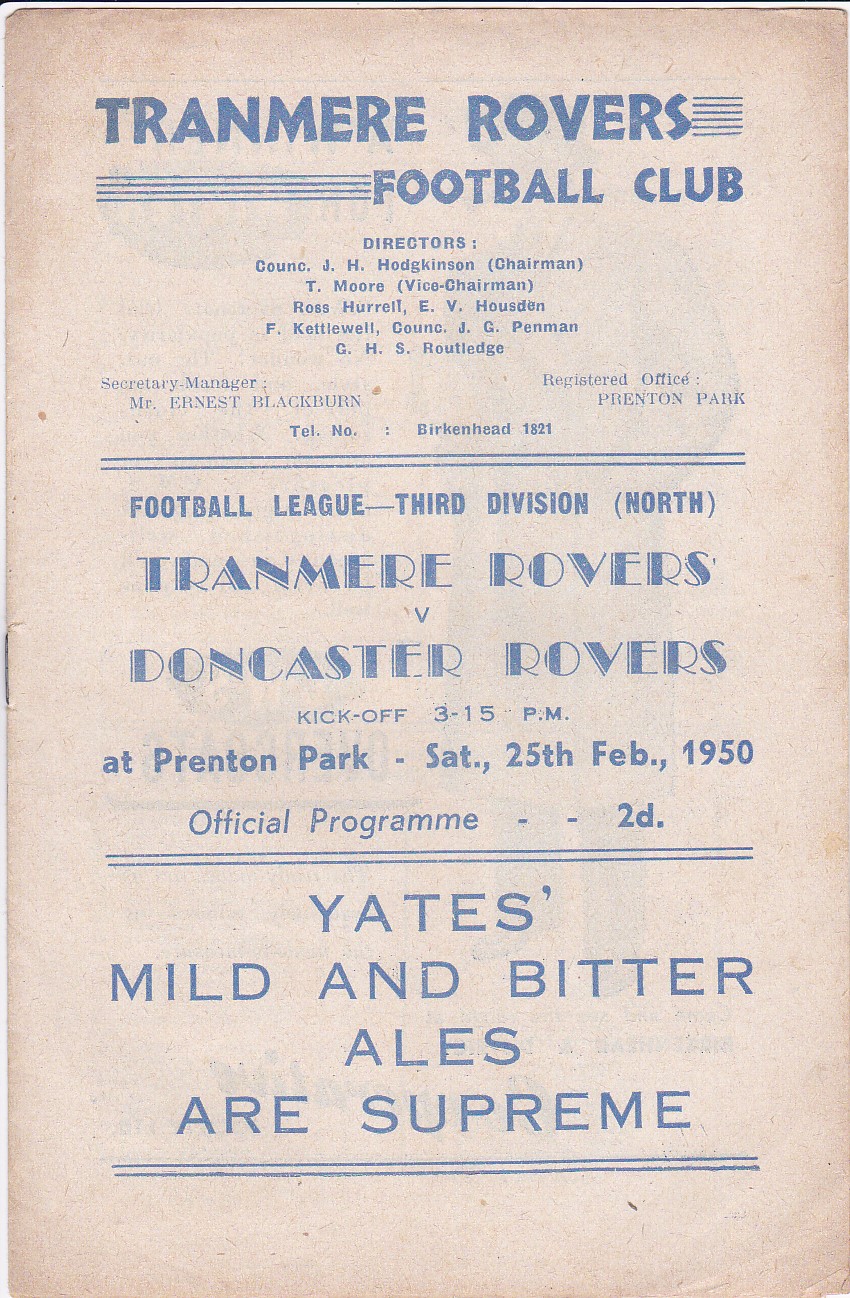This image displays an old and faded sports program for a Tranmere Rovers football match, printed on an ivory background with text in a faded blue. At the top, it prominently features "TRANMERE ROVERS FOOTBALL CLUB" in all capitals. Beneath that, it lists the directors: J.H. Hodgkinson (Chairman), T. Moore (Vice Chairman), Ross Hurrell, E.V. Woodson, F. Cuttlewell, J.G. Penman, and C.H.S. Rutledge, with the secretary-manager Mr. Ernest Blackburn. The registered office is listed as Prenton Park with the telephone number Birkenhead 1821. Below, flanked by two thin blue lines, the program announces the football league third division North match between Tranmere Rovers and Doncaster Rovers, scheduled to kickoff at 3:15 p.m. at Prenton Park on Saturday, 25th February 1950. It states "Official Program - 2d" and at the bottom declares in large letters, "Yates' Mild and Bitter Ales Are Supreme," accompanied by additional blue lines. A visible staple on the left edge hints at the program's age and structure.